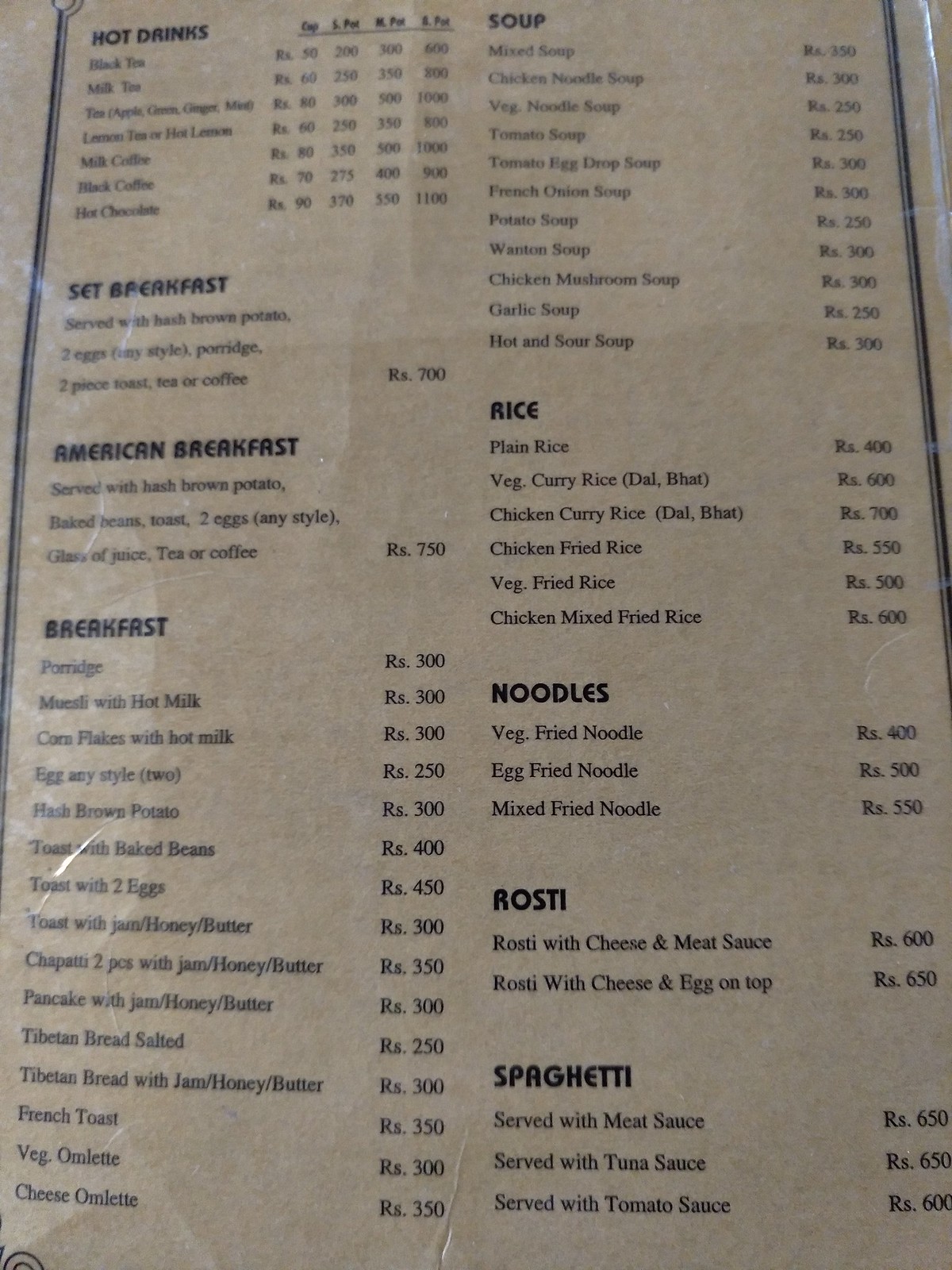**Descriptive Caption:**

"This image displays an extensive restaurant menu, starting with a section for hot drinks which includes options such as Black Tea, Milk Tea, Chai Tea, and Hot Chocolate. The breakfast offerings are divided into various sections: 

- Basic Breakfast: Two eggs cooked in any style, served with porridge and two pieces of toast, accompanied by tea or coffee for $7.
- American Breakfast: A more substantial option featuring hash brown potatoes, baked beans, two eggs any style, a glass of juice, and tea or coffee for $7.50.

Additional Breakfast Menu Items:
- Porridge
- Muesli with hot milk
- Cornflakes with hot milk
- Eggs any style
- Hash brown potatoes
- Toast with baked beans
- Toast with two eggs
- Toast with jam, honey, and butter
- Shabbiri: Two pieces served with jam, honey, and butter
- Pancakes: Served with jam, honey, and butter
- Tibetan bread (salted) with jam, honey, and butter
- French toast
- Veggie omelet
- Cheese omelet

The menu also details a variety of soup options:
- Mixed Soup
- Chicken Vegetable Soup
- Tomato Soup
- Tomato Egg Drop Soup
- French Onion Soup
- Potato Soup
- Wonton Soup
- Chicken Mushroom Soup
- Garlic Soup
- Hot and Sour Soup

In addition to these sections, the image hints at several more items available, promising a comprehensive dining experience."